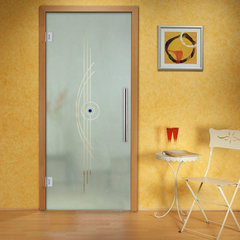This photograph captures the interior of a room with a modern yet cozy home decoration style. Central to the image is a grey door with a large handle on its left side; the door is framed in brown wood and has a gold semi-transparent design down the middle, featuring intricate patterns of straight and curved lines intersecting a circle with a blue dot. The walls surrounding the door are a warm yellow, enhancing the inviting atmosphere of the space. Adjacent to the wall on the right side of the image, there’s a small circular white table accompanied by a similarly colored white chair. Upon the table are two tall glass cups filled with a red liquid. Above this arrangement hangs a square abstract art piece with a white frame, the artwork itself predominantly yellow with a dark ring, a white intersecting line in one corner, and a distinctive red splotch. The floor is a rich brown hardwood, adding a touch of elegance to the room. The overall composition of the space suggests a comfortable and stylish living area.